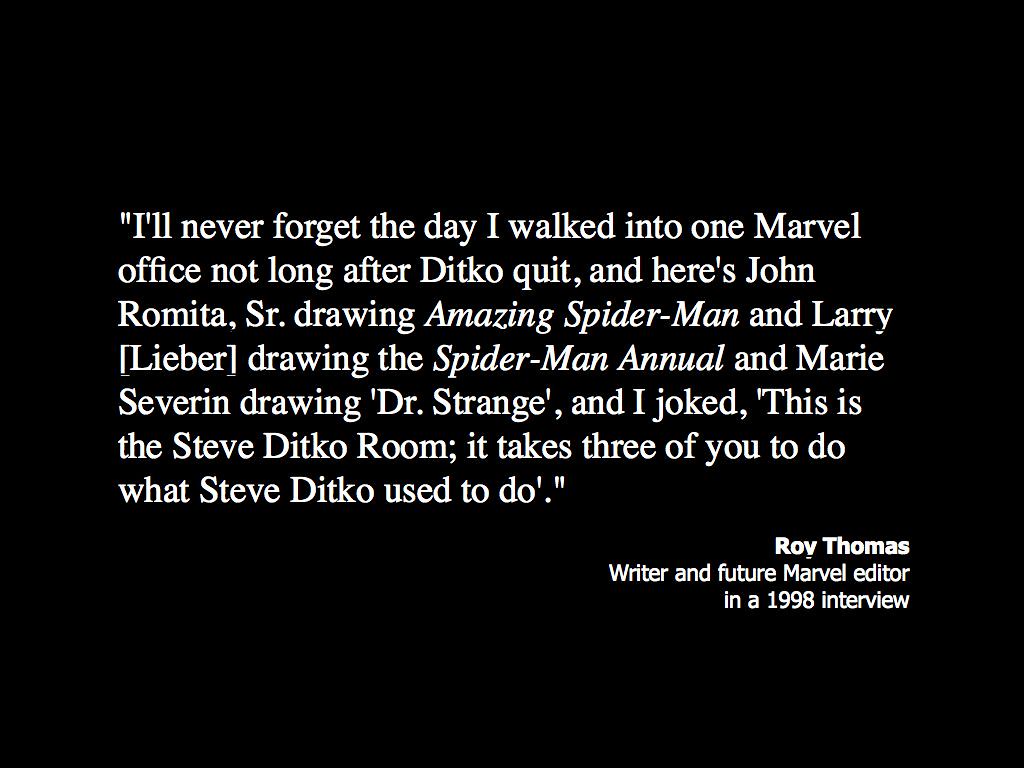The image features a quote on an 8-inch by 8-inch black background with white text centered in the middle, leaving a large margin around the top, bottom, left, and right sides. The quote reads: "I'll never forget the day I walked into one Marvel office not long after Ditko quit. And here's John Romita Sr. drawing Amazing Spider-Man and Larry Lieber drawing the Spider-Man annual and Marie Severin drawing Doctor Strange. And I joked, this is the Steve Ditko room. It takes three of you to do what Steve Ditko used to do." The attribution, right-aligned below the quote, states: "Roy Thomas, writer and future Marvel editor, in a 1998 interview."